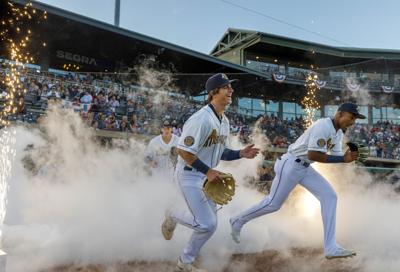In this vibrant daytime photograph, a pair of exuberant baseball players race onto the field amidst a festive haze of smoke and golden confetti, their white uniforms accentuated by blue caps. One, an African American player, sports a black mitt, while his white teammate carries a brown mitt. Behind them, closer to the cheering crowd in the stands, another player begins to emerge through the celebratory smoke. The stadium, adorned with the inscription "Segra" on the bleachers, gives off a smaller, possibly minor league vibe, with its greenish, wooden structure filled with enthusiastic fans. Flames and sparkler-like pyrotechnics add to the jubilant atmosphere, as the vivid blue sky overhead encapsulates the scene.